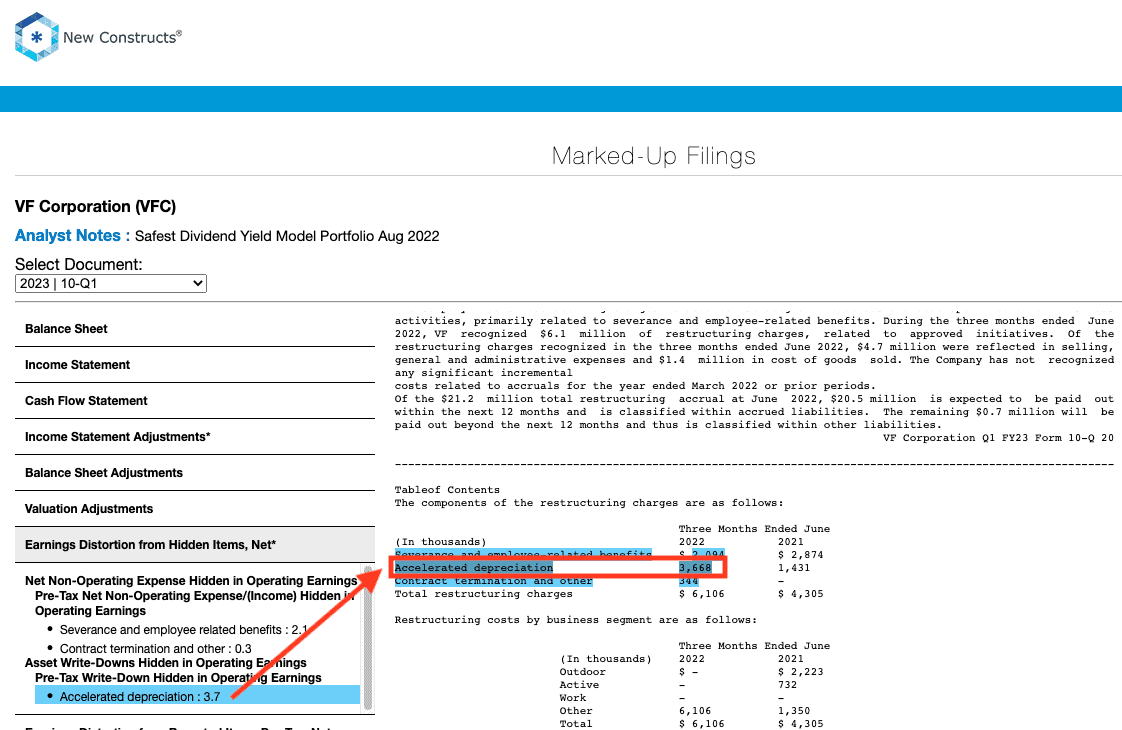The image displays a web page from the "New Constructs" website, featuring financial information and analyst notes. At the top left corner, the "New Constructs" logo is prominently visible. Directly below the logo, there is a long blue bar. Beneath the blue bar, in black and white text, is the heading "Marked Up Filings." Under this section, the title "VF Corporation" is presented, followed by a subheading: "Analyst Notes Safest Dividend Yield Model Portfolio August 2022."

Further down, there is a dropdown menu labeled "Select Document," which offers various options including "Balance Sheet," "Income Statement," "Cash Flow Statement," "Income Statement Adjustments," "Balance Sheet Adjustments," "Valuation Adjustments," and "Earning Distortion from Hidden Items Net."

On the right side of the page, smaller font text provides detailed information about VF Corporation's restructuring activities. It explains that activities related primarily to severance and employee-related benefits resulted in VF recognizing $6.1 million in restructuring charges during the three months ending June 2022. Of these charges, $4.7 million were included in Selling, General, and Administrative expenses, and $1.4 million were accounted for in the Cost of Goods Sold.